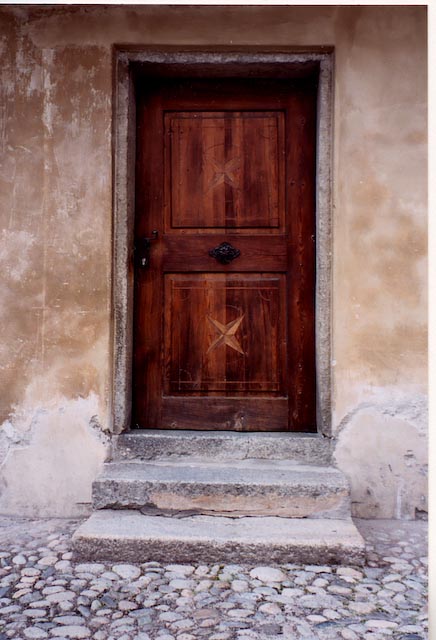The image captures a vertically aligned rectangular photograph of an antiquated structure, possibly a house, prominently featuring its dark brown wooden door centered in the scene. This door, which is adorned with two star-shaped insignias on the top and bottom panels, also displays a metallic medallion in the middle. The door is complemented by a black handle situated on the left side. Surrounding this door is a worn stone wall with weathered cement plaster or stucco, streaked with white and beige tints especially noticeable in the upper left-hand area. Leading up to the door are three aged, gray stone steps, flanked by a walkway composed of large, gray and white pebbled stones. This entire scene exudes an architectural style likely uncommon in America, with an unmistakable historical and foreign charm.